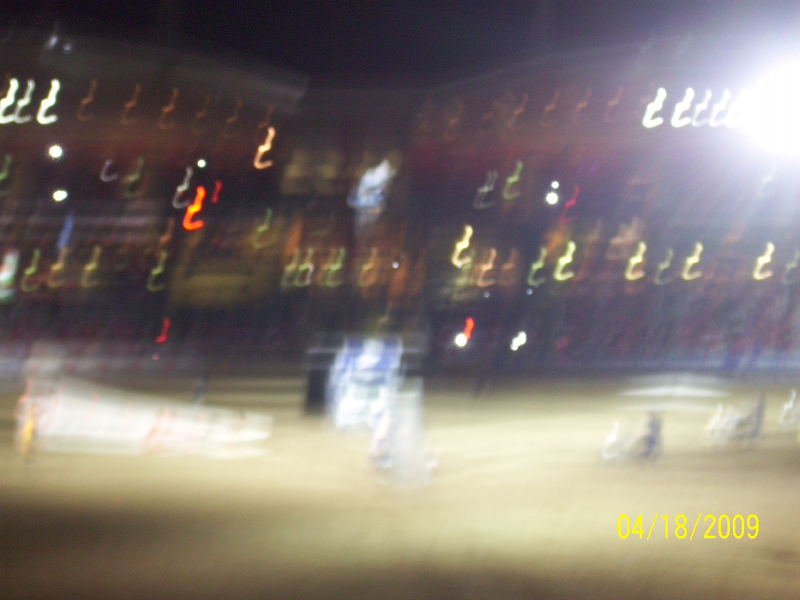The image is somewhat blurry, evoking an initial impression of a rodeo, though no clear signs of bulls are present. Central to the composition is a person standing on a podium, dressed in a white shirt, extending their left arm toward the viewer. Surrounding this focal figure is a series of objects resembling baby carriages or buggies, with three clearly visible and part of a fourth just discernible on the right. The center of the image features a vague white shape with a blue item, marked by a white dot, trailing behind it. Adjacent to this is another white object positioned horizontally. In the background, rows of bleachers are partially visible, illuminated by lights suspended above, their shapes reminiscent of inverted question marks. These lights glow in a spectrum of colors including yellow, green, pink, orange, and blue. The foreground ground appears tan in hue, suggesting a sandy surface.